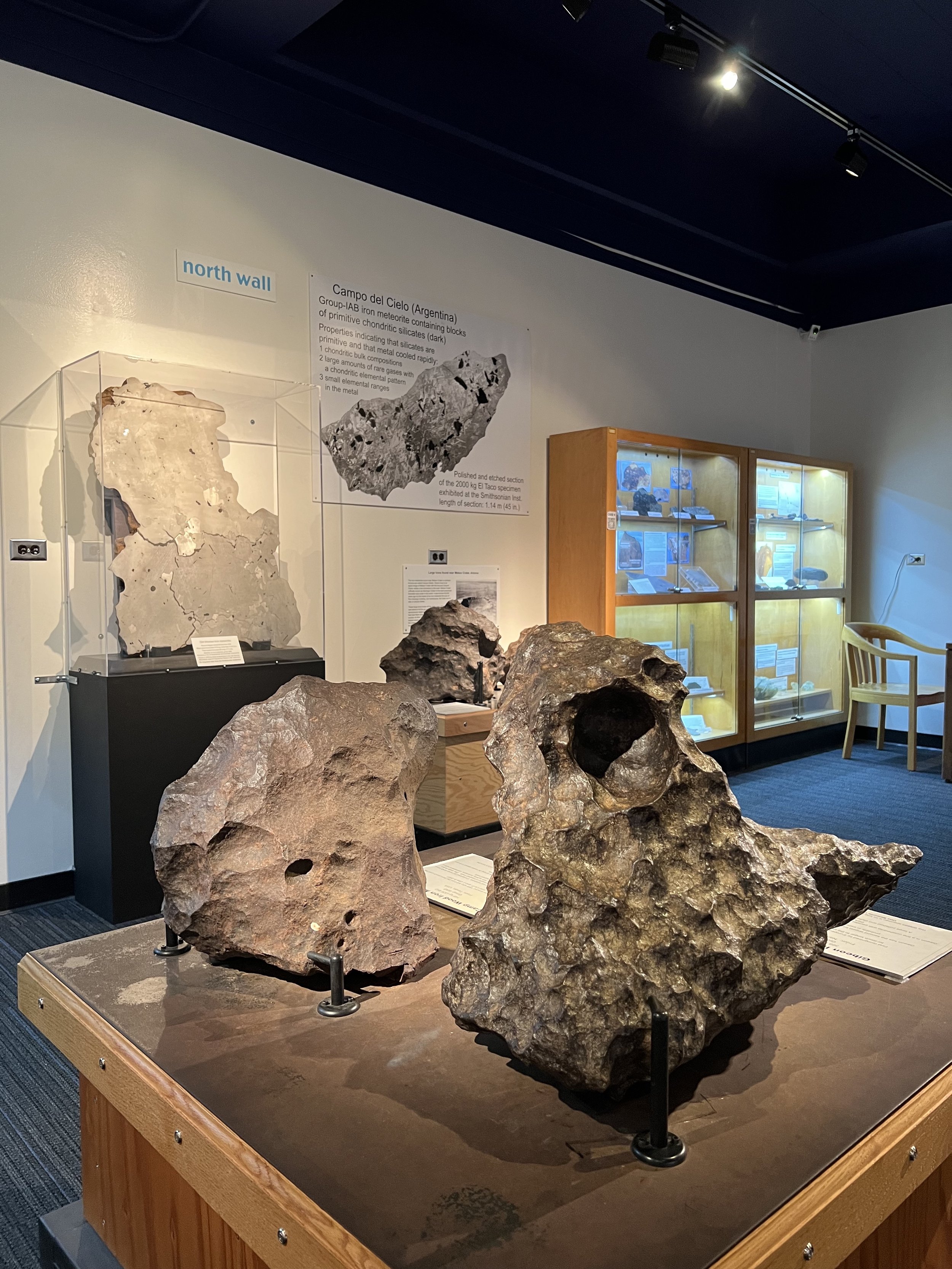Inside a museum, the image showcases a detailed and organized display of rock exhibits. Dominating the scene are several glass display cases, each containing various labeled items, although the specific labels are too small to discern. In the foreground, a table presents two substantial rocks mounted on posts amidst an array of informational displays that are difficult to read from the image. The rocks, possibly meteorites given their cratered appearance, are accompanied by a dark gray pedestal with a light wood base. 

The backdrop features a black ceiling equipped with strategic lighting, white walls adorned with photographs and descriptions related to rocks, and a gray carpeted floor. Particularly notable is a section labeled "North Wall," distinguished by a white and blue sign. Adjacent to this is a poster labeled "Campo del Cielo, Argentina," hinting at the origins of the meteorites on display. Further to the right, a large glass cabinet houses a substantial rock piece, potentially a stone table from ancient times, illuminated by internal lighting. A nearby wooden chair and an outlet with a white cord add functional context to the setting. The overall color palette captures tones of white, blue, black, gray, and hints of yellow, contributing to a visually cohesive and informative exhibition space centered around geological specimens and ancient artifacts.